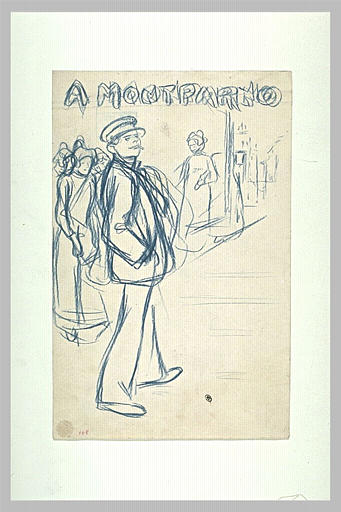This detailed sketch on what appears to be an aged, off-white paper is meticulously framed with a white cardstock and a gray outer frame. The drawing, executed in dark blue or black pencil, showcases a vivid outdoor scene. Central to the composition is a man wearing a long-sleeve sport jacket and a cap, resembling a conductor's or sailor's hat. His casual stance with one hand in his pocket and the other possibly holding a cigarette adds a touch of realism. The text at the top reads, "Ah, Mount Matra" or possibly "A. Montparno," though the exact wording is unclear.

To the left behind the man, there is a woman in a long dress with a shawl or bonnet over her head, looking downward. To the right, another woman in a long dress is captured in motion, walking towards the man while holding an indistinguishable object. The background subtly hints at the presence of a street sidewalk and faint outlines of buildings, reinforcing the outdoor setting. The overall scene is rendered with a light touch, giving it a delicate and somewhat nostalgic feel.